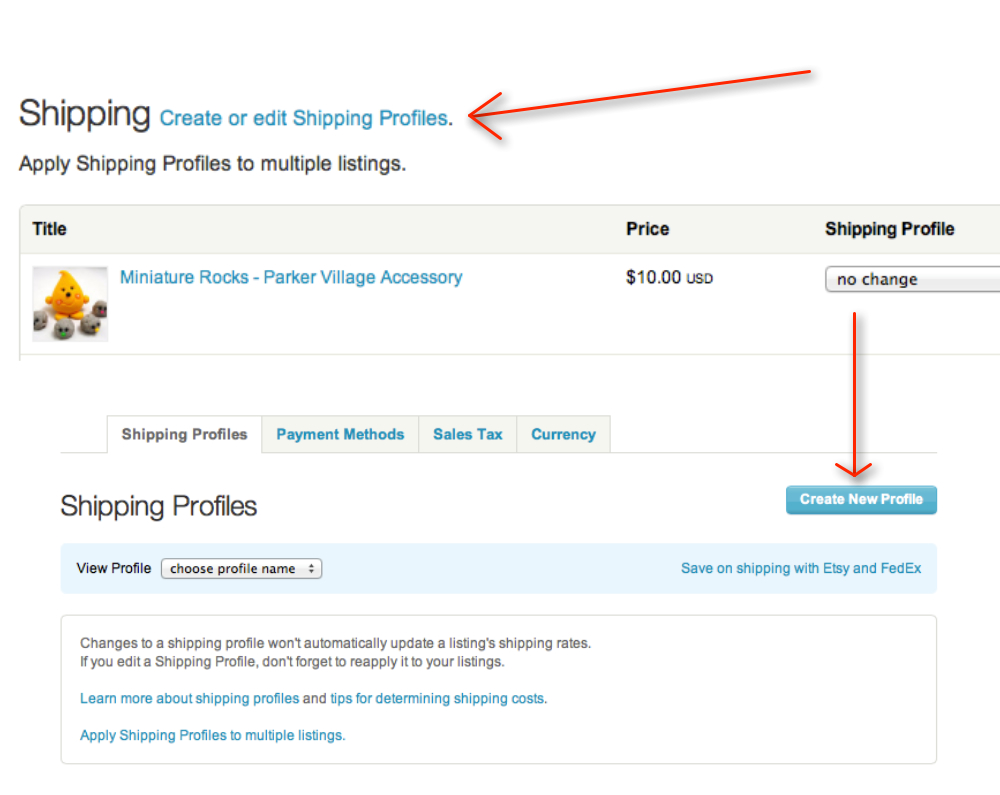This image features a detailed screenshot of an e-commerce website interface designed for selling various items. Prominent red arrows draw attention to key areas, providing guidance on shipping configurations. The first arrow directs towards the top of the page, highlighting the section labeled "Create or edit shipping profiles." Below this, another arrow points to instructions on how to "Apply shipping profiles to multiple listings."

In the main section of the screenshot, there is a listing for a product titled "Miniature Rocks, Parker Village Accessory," accompanied by an image of a small, decorative rock item. The price of the item is visible, and a section labeled "Shipping Profile" is displayed with a dropdown menu set to "No Change." Another red arrow transitions from this dropdown towards the "Create New Profile" prompt, indicating the option to define a new shipping profile.

At the bottom of the image, the interface contains tabs labeled "Shipping Profiles," "Payment Methods," "Sales Tax," and "Currency," indicating various configuration options available to the seller.